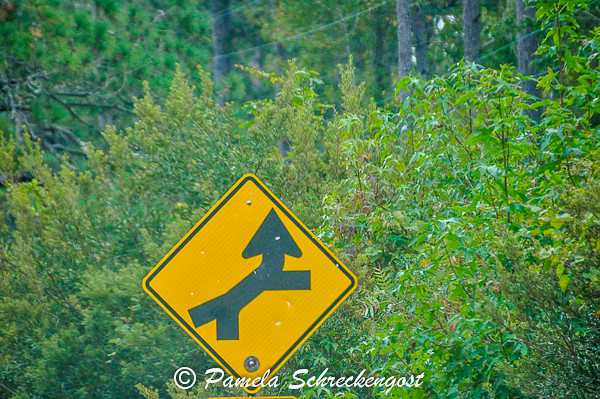This photograph captures a classic yellow diamond road sign with a black border prominently positioned in the foreground. The sign features a complex arrow design: the arrow curves from the left, sweeps upwards, and then turns vertical just past the center. From the bottom left area, another mirrored arrow emerges, creating an impression of two paths that merge initially and then split again. At the bottom of the sign, the elegant cursive text reads "copyright Pamela Schreckengast."

The background offers a serene woodland scene, predominantly covered by green foliage and featuring several tree trunks, including a cluster of three close together and another set a bit farther away, extending off the top of the image. Amidst the greenery, some tall pine trees and a mix of light and dark green foliage add texture to the scene. There are also visible lines in the background, possibly phone or power cables, stretching across the forested landscape. The photograph captures a sunny day, enhancing the vibrant greens and the detail of the forest background. Additionally, a glimpse of another sign beneath the main diamond-shaped one is visible, revealing only the yellow color and a bit of its border.